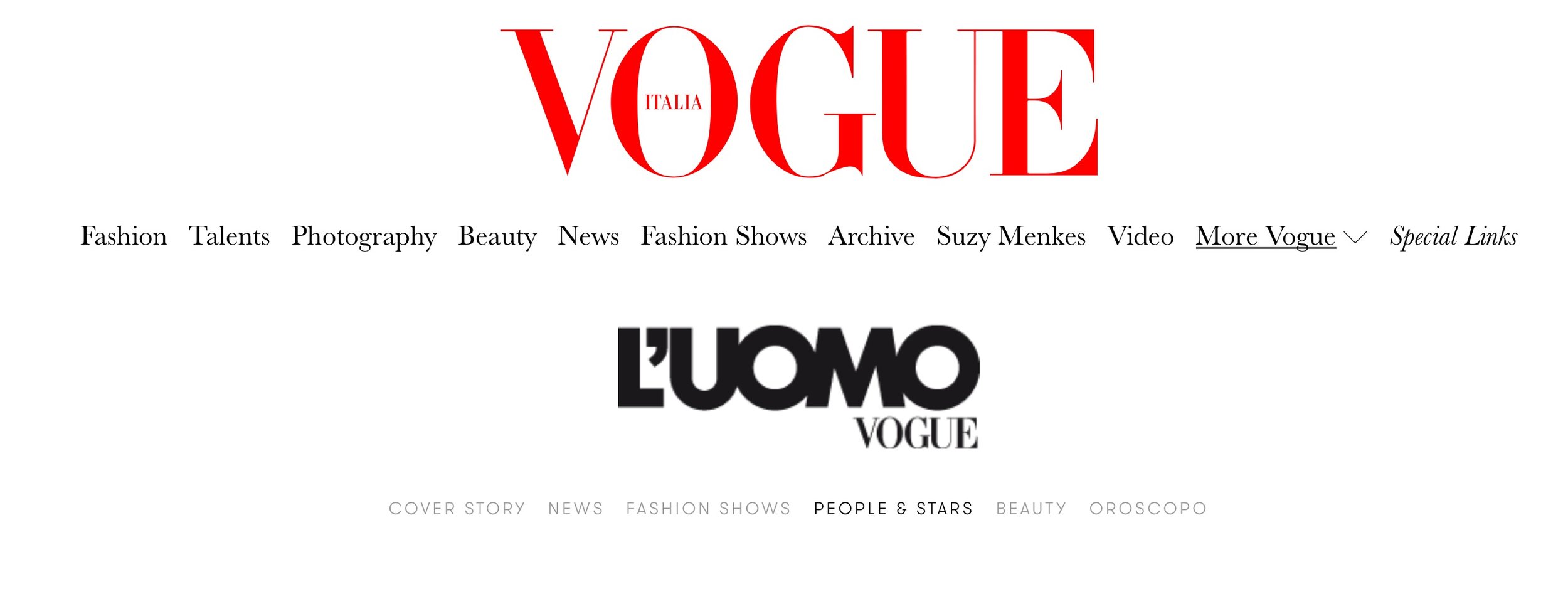The image displays the homepage of the Italian Vogue website prominently. At the top of the webpage, the iconic "VOGUE" logo is presented in large, bold red letters. Positioned within the letter "O" is the word "Italian" indicating the specialized edition. The site features a horizontal navigation bar with several clickable links categorized from left to right: Fashion, Talents, Photography, Beauty, News, Fashion Shows, Archives, Zuzi Minx, and Video. An additional link labeled "More Vogue" with a downward-pointing arrow offers access to further features. A "Special Links" button is included as well. At the bottom of the page, "L'UOMO Vogue" is boldly printed in black, signifying the men's edition of the magazine. In very small print at the very bottom of the screen are additional navigation links: Cover Story, News, Fashion Shows, People and Stars, Beauty, and Auroscopo.